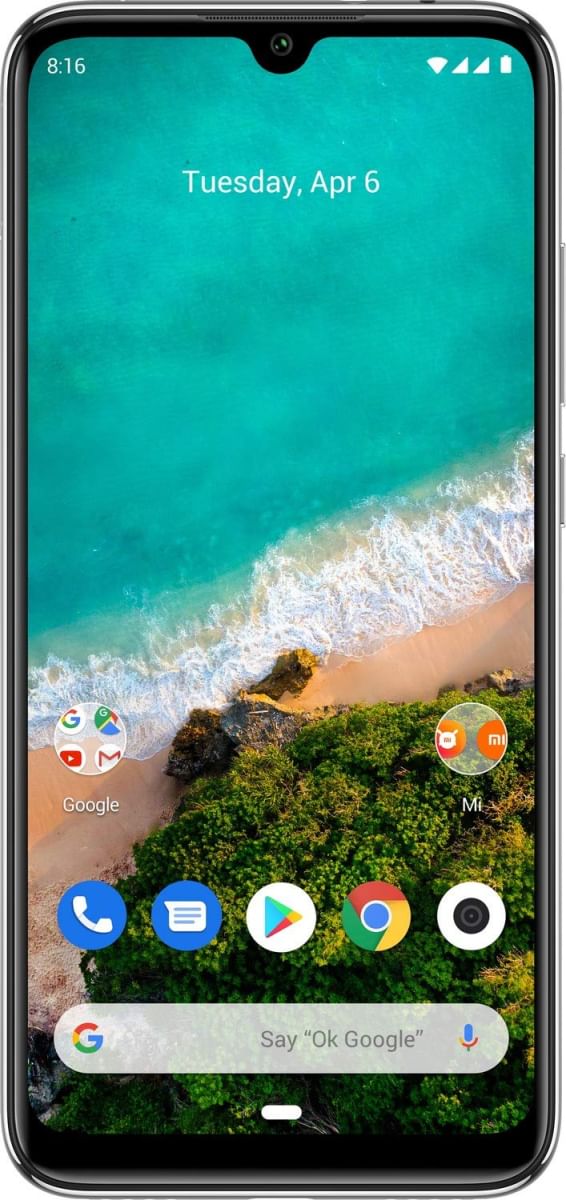The image displays the front of a smartphone with a beach-themed wallpaper. At the top of the screen, it's 8:16 AM, indicated alongside icons including a signal triangle, what might be a slice of pizza symbol, two triangles, and a battery indicator. Between the time display and the icons, there is a small camera. Below this, the screen shows the date: Tuesday, April 6th. 

Further down, there are two app folders: one labeled "Google" containing various Google apps, and another labeled "MI" with additional unspecified apps. At the bottom of the screen, there are individual app icons for phone calls, messaging, the Google Play Store, Google search, and possibly the camera. Beneath these icons is a Google search bar, featuring the "G" logo, an "OK Google" prompt, and a microphone icon.

The phone itself has a black bezel surrounding the display, and the outer edge of the device appears to be silver. The beach scene wallpaper showcases a green ocean with waves breaking on the shore, stretching from the top of the screen to about halfway down. The image is angled and includes a sandy beach with rock outcroppings, adorned with patches of greenery, about two-thirds down the left side of the screen.